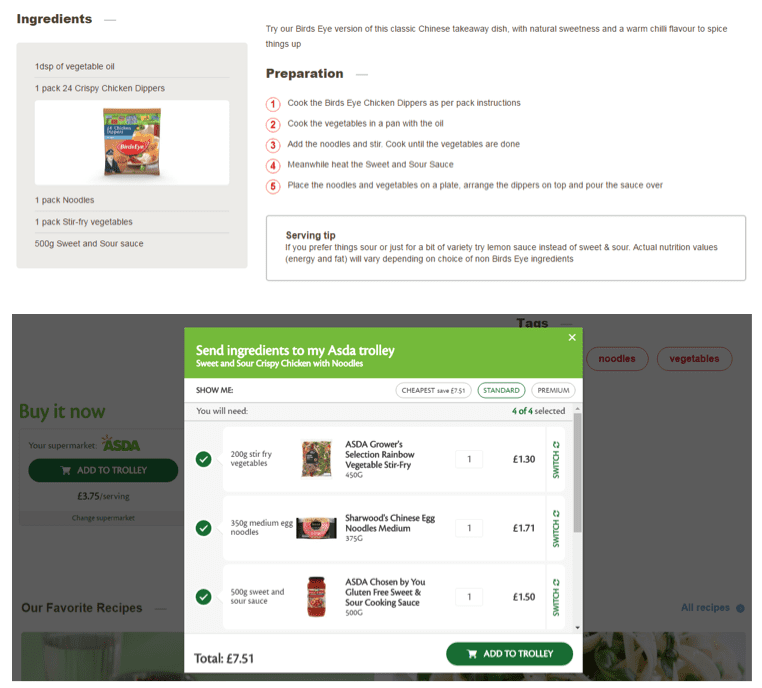The image showcases a cooking website featuring a recipe for Sweet and Sour Chicken Crispy Noodles. In the upper left-hand corner, the word "Ingredients" is prominently displayed in dark black font. Directly below, a gray box lists the necessary components for the dish: one teaspoon of vegetable oil, one pack of 24 crispy chicken dippers, one pack of noodles, one pack of stir-fry vegetables, and 500 grams of sweet and sour sauce. 

The description suggests trying their Bird's Eye version of the classic Chinese takeaway dish, noted for its natural sweetness and a touch of chili for added spice. 

Next, large letters spell out "Preparation," beneath which the cooking steps are neatly listed in sequential order, marked by red, circular numbers from one to five. 

A serving tip advises that if a sourer taste is preferred or for some variety, lemon sauce can be used in place of the sweet and sour sauce. It also mentions that actual nutritional values, energy, and fat content may vary depending on the choice of ingredients not from Bird's Eye.

Additionally, there is a pop-up page in the background that reads "Buy It Now." It includes an "Add to Trolley" button, indicating that this is likely a non-American website, as "trolley" is the term used in some countries. The page allows users to send the listed ingredients directly to their trolley, essentially a wish list, for purchase. Prices for each ingredient are displayed, and a green bar at the bottom provides the option to "Add to Trolley."